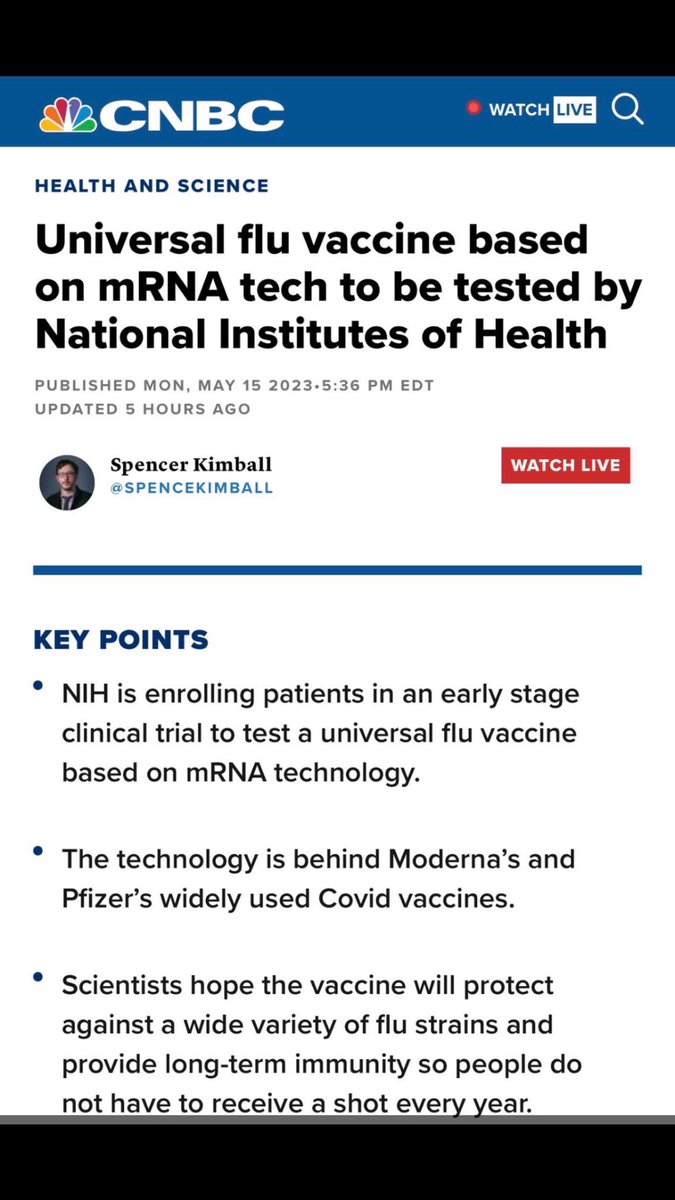The image features a dark blue header at the top, bordered by a black strip above it. Within this blue section is the NBC logo alongside the text "CNBC" and "Watch Live." Below this, the text reads "Health and Science: Universal Flu Vaccine Based on mRNA Tech to be Tested by National Institutes of Health," which was published on May 19th, 2023, at 5:36 PM EDT and updated five hours ago by Spencer Kimball. 

Following this, there is a "Key Point" section with bullet points highlighting that the NIH is enrolling patients in an early-stage clinical trial to test a universal flu vaccine using mRNA technology, the same technology behind Moderna and Pfizer's COVID-19 vaccines. The objective is to create a vaccine that protects against multiple flu strains and provides long-term immunity, reducing the need for annual flu shots.

At the bottom of the image, there is a black rectangular box.